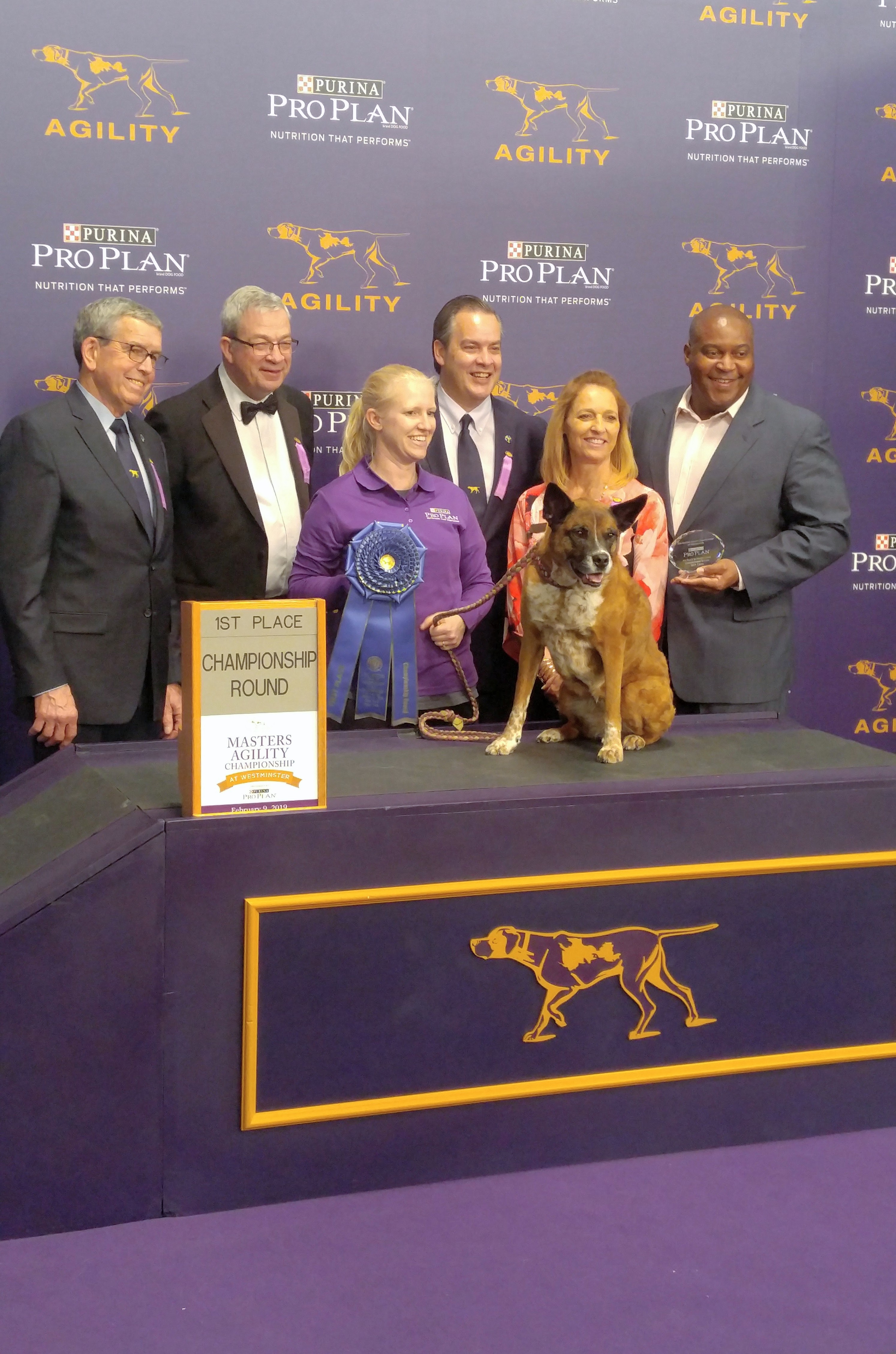The photograph captures an indoor dog show, specifically an agility competition, with a prominent background featuring a repeating pattern of the Purina ProPlan logo and their slogan, "Nutrition that performs," alongside a yellow silhouette of a pointing dog with the word "Agility." In the center of the image, six individuals stand around a unique, green, brown, and purple long-shaped desk adorned with a striped dog silhouette. The group includes a black man, two white women, and three white men, all appearing to be judges or officials. 

One of the women, dressed in a purple shirt, is proudly holding a blue ribbon and the leash of a brown and white dog with dark brown ears, which stands on the desk. The well-groomed dog, the star of the show, gazes directly into the camera. To the left of the dog, a small placard reads "First Place Championship Round Masters Agility," commemorating the dog's victory. The ground beneath the desk is covered in purple carpeting, adding to the formal, celebratory atmosphere of the event.